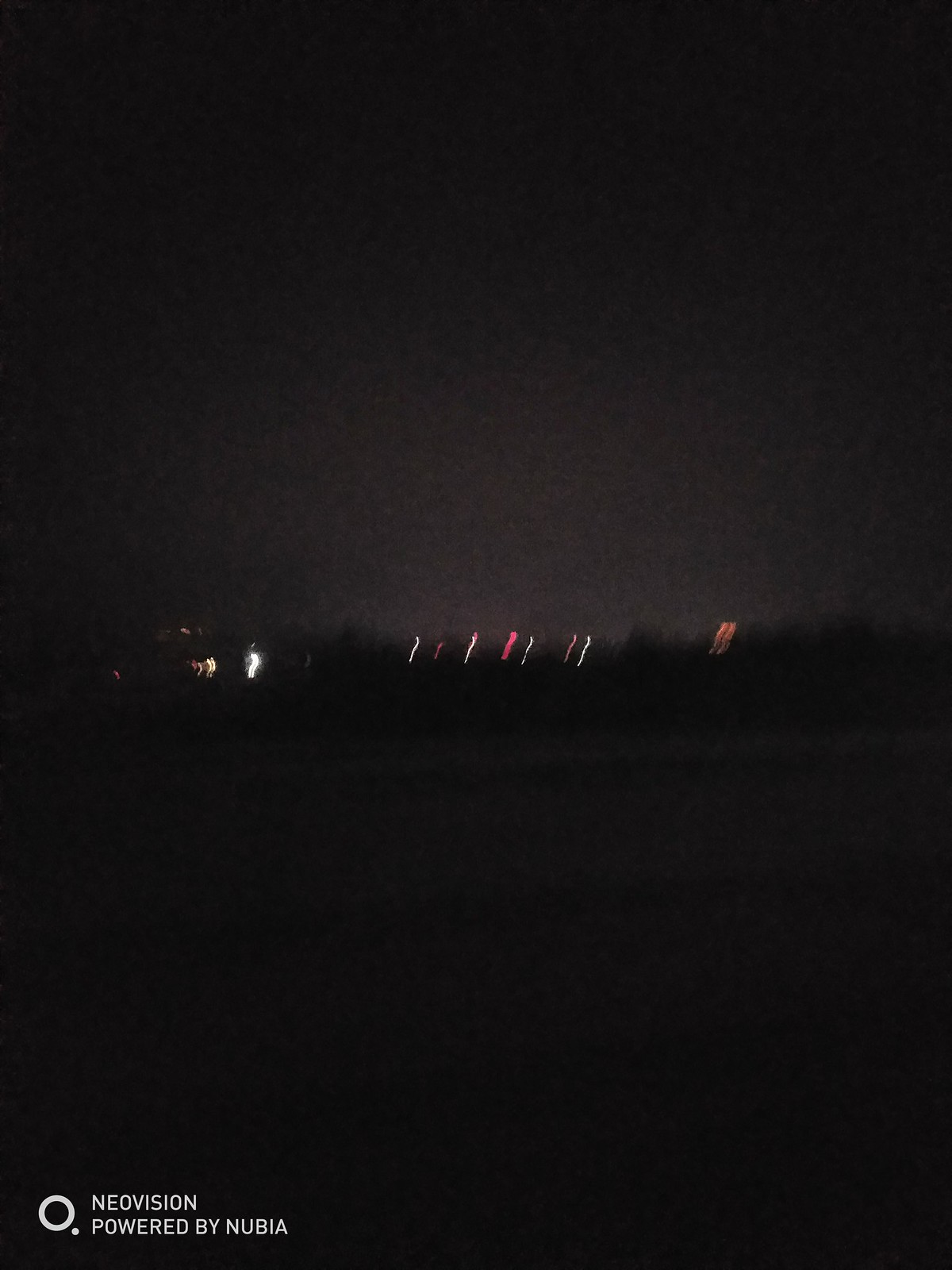This photograph, taken outside at night, is dark and very blurry, making it hard to distinguish specific details. The foreground is a mix of dark gray shades, and the horizon features a tree line with barely visible lights. The lights along the horizon appear as streaks due to motion blur, and they are a mixture of red, white, and yellow, possibly from vehicle headlights and taillights. The background comprises a hazy, indistinct glow, perhaps from distant city lights or buildings. No moon or stars are visible in the night sky. There is also a noticeable text at the bottom left corner, with the inscription "NeoVision powered by Nubia" alongside a white circle and dot.